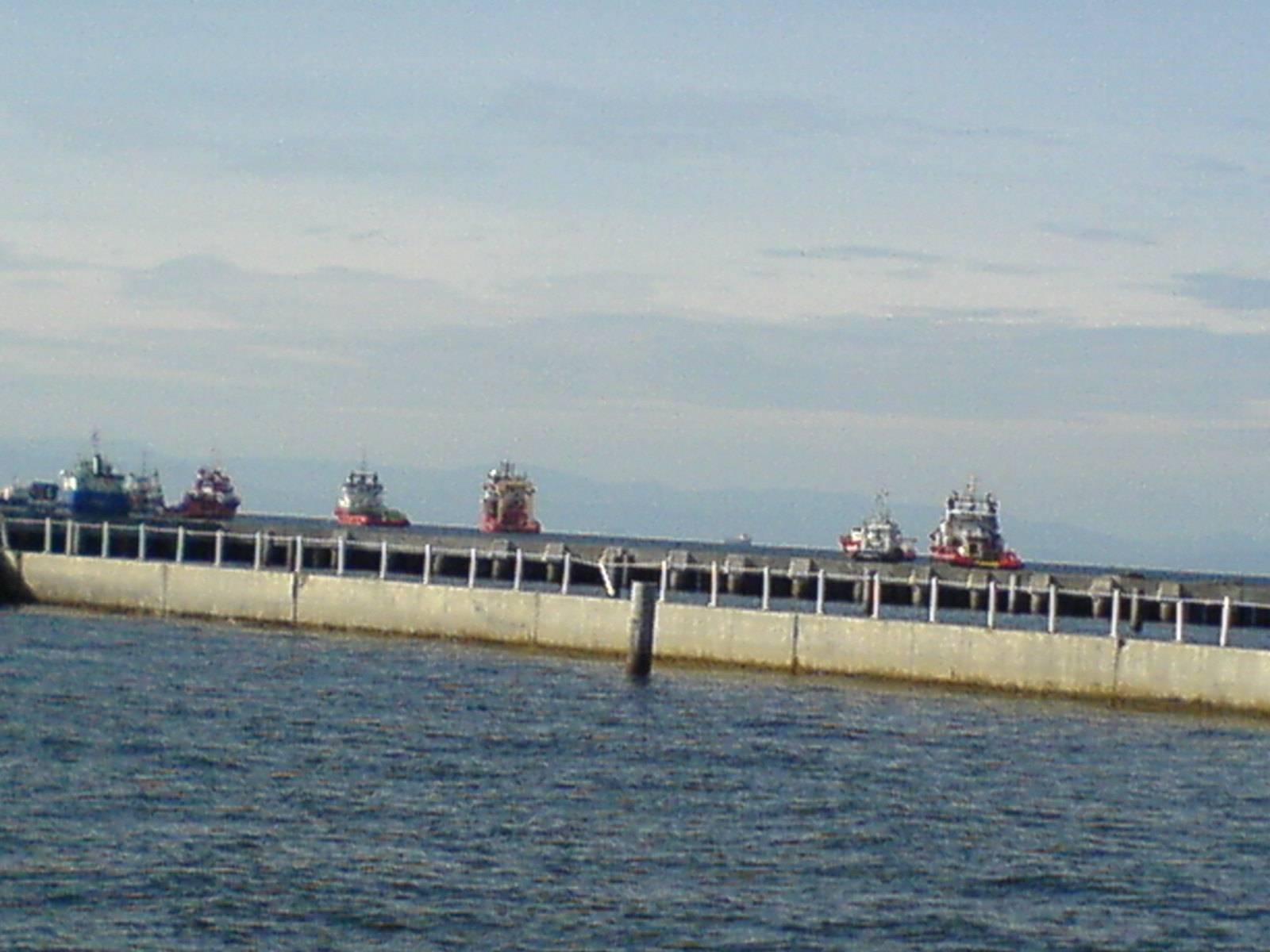The image captures a serene yet intricate maritime scene. In the foreground, a concrete breakwater wall extends through the bay area, safeguarding against stormy conditions. A black pipeline with multiple joints runs along this light grey concrete platform, bordered by a silver fence. A vertical pipe stands prominently near the wall. The calm, blue sea spreads out on either side, with gentle waves marking its surface. The sky above is overcast with low-hanging, dark grey clouds lingering under a light blue and white canopy.

In the distance, several boats of various sizes are visible. These vessels, primarily red and white, include one blue and white boat and a brown and red one. Among these, some boats stand closer while others appear as small dots on the horizon. The ships are commercial in nature, possibly fishing or cargo boats, featuring smokestacks or tall instrumentation. Beyond the fleet of boats, either mountainous terrain or thick cloud cover forms the distant backdrop, rounding off the tranquil maritime vista.